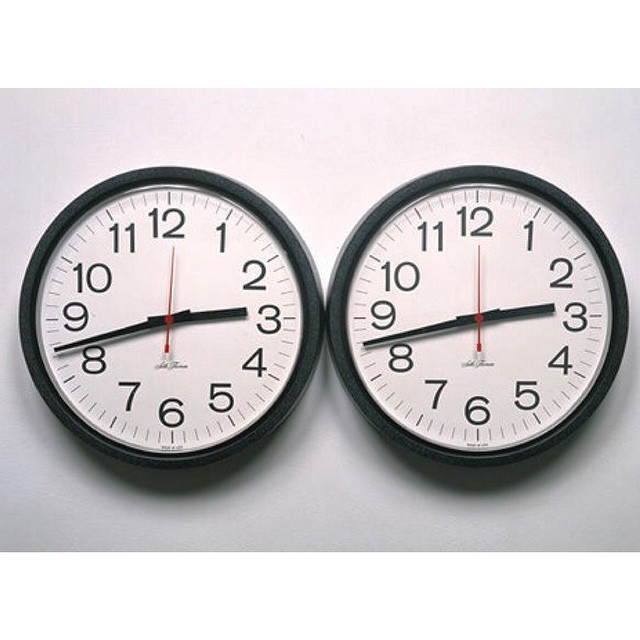This is a color photograph depicting two nearly identical round wall clocks positioned side by side, just touching. The background is grey and gradually becomes lighter towards the top, with some shadows cast toward the bottom. A light source from above creates slight shadows underneath the clocks. Both clocks have a thick black frame with a potential silvery reflection underneath it. The clocks feature large black numbers from one to twelve, with smaller notches indicating the minutes. Every five-minute line is bolder than the minute lines in between. The clocks have a black hour hand, a black minute hand that is tapered, and a thinner red second hand. The faces of the clocks are white, and there is a tiny, unreadable cursive logo or signature at the center below the hands. The time displayed on both clocks is approximately 2:43, though the second hand on the clock to the left is slightly ahead by one second, situated just past the 12, while the second hand on the clock to the right is exactly at the 12.